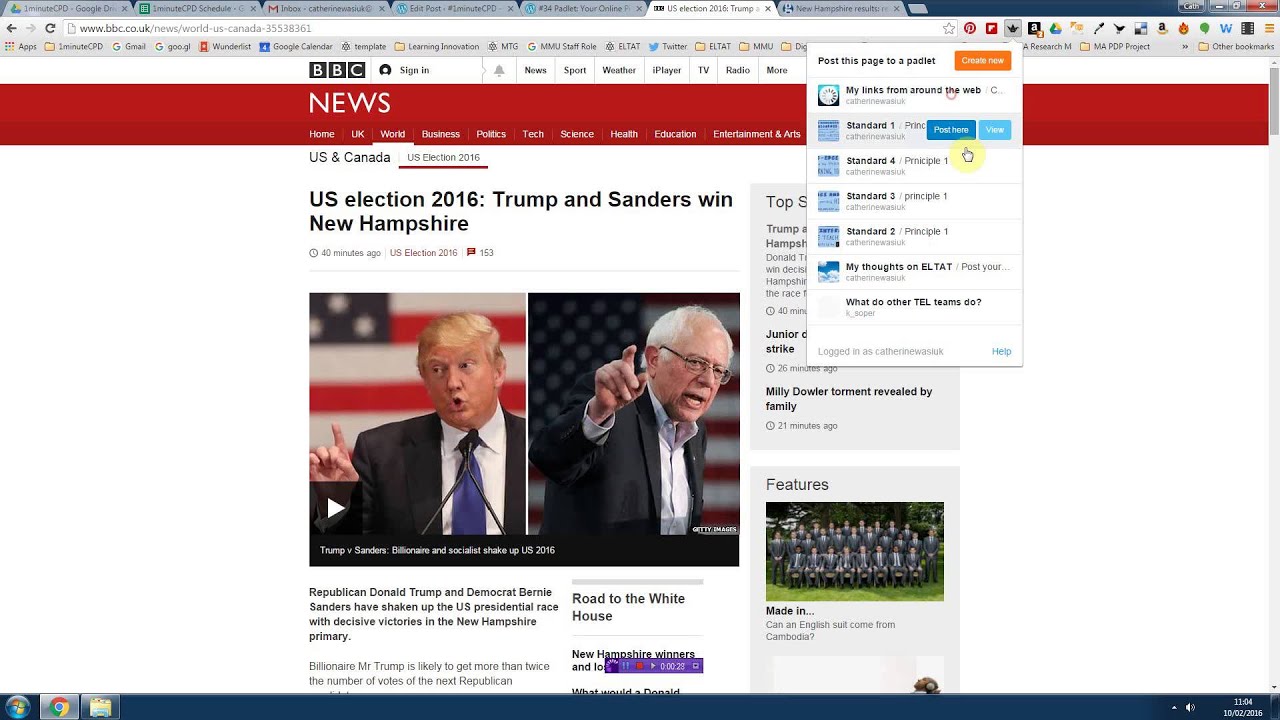This image is a screenshot captured from a computer monitor displaying the BBC News website. The web browser currently has seven tabs open, with the active tab being for BBC News. The top navigation bar on the BBC News website features several tabs including Sign In, Notifications, News, Sports, Weather, iPlayer, TV, Radio, and More. The prominent red BBC banner is visible, featuring additional navigation options such as Home, UK, World, Resources, Politics, Tech, Service, Health, Education, Entertainment, and Arts.

Beneath the main navigation, there is a white section highlighting two specific categories: U.S. & Canada and U.S. Election 2016. Below this is another red BBC News bar, under which the main headline reads: “U.S. Election 2016: Trump and Sanders win New Hampshire.” The article features photographs of Donald Trump and Bernie Sanders, both in front of American flags and appearing to be in mid-speech or gesture.

The accompanying text beneath the headline states: "Republican Donald Trump and Democrat Bernie Sanders have shaken up the U.S. presidential race with decisive victories in the New Hampshire primary." The screenshot captures the beginning of a detailed article on their primary wins. The site clearly displays the content alignment and visual structure typical of BBC News Online.